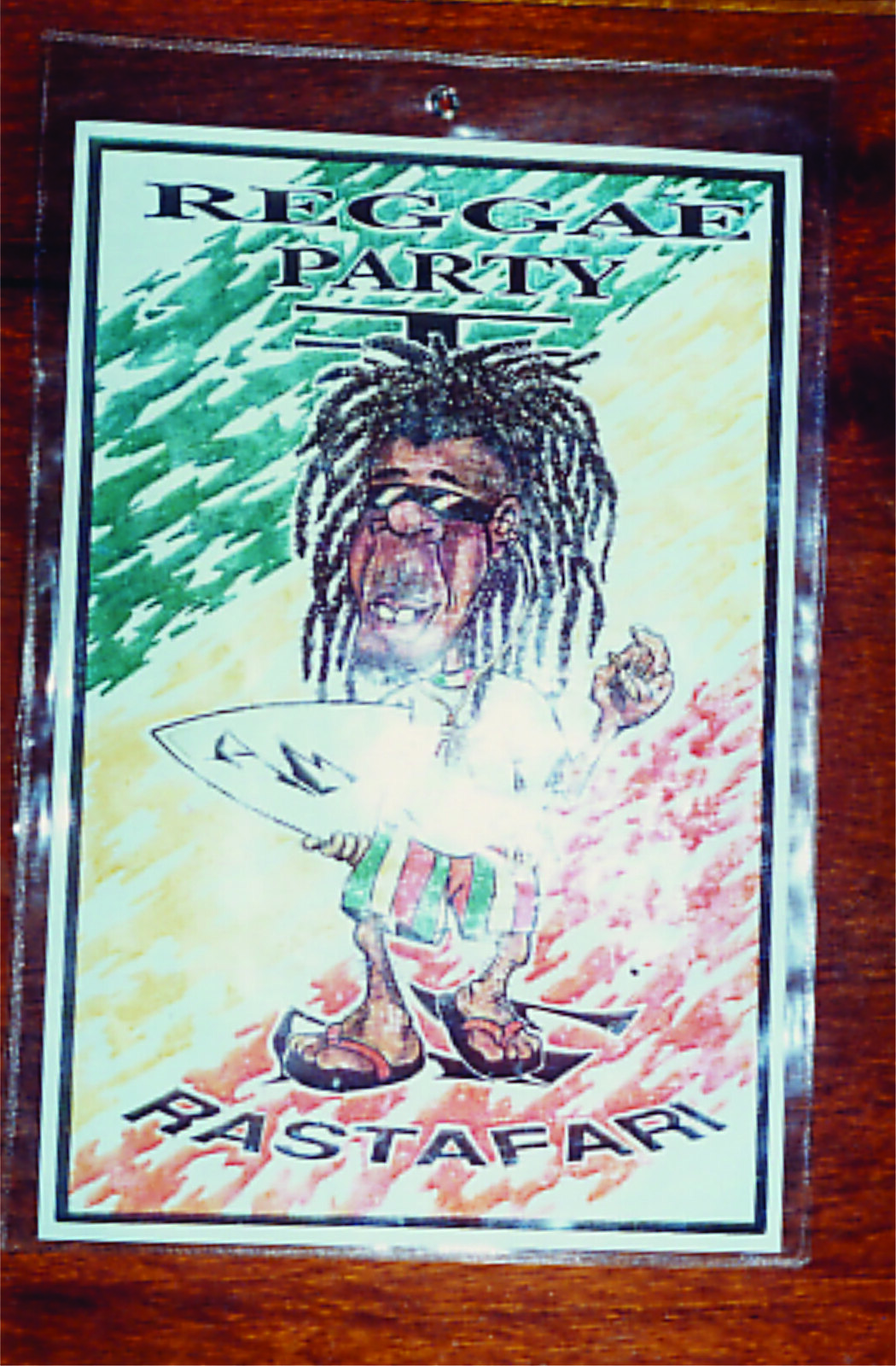This image depicts a laminated poster on a wooden table or wall, enclosed in a clear plastic protector. The poster features a lively and colorful illustration with a background of striped green, yellow, orange, and white. At the top, bold black letters spell out "Reggae Party," clearly inspired by the reggae genre, and at the bottom, it reads "Rastafari" in capitalized bold black letters.

The central figure is a caricature of a Jamaican man, reminiscent of Bob Marley, donning long dreadlocks and dark sunglasses. He is dressed in striped green, white, and orange swim shorts, and orange-strapped sandals or flip flops. The character exudes a laid-back vibe, standing on a towel, smoking a joint, and holding a triangular object that might be a surfboard. The illustration has a beachy background, possibly depicting waves and sand, enhancing the chill, reggae beach party theme of the poster.